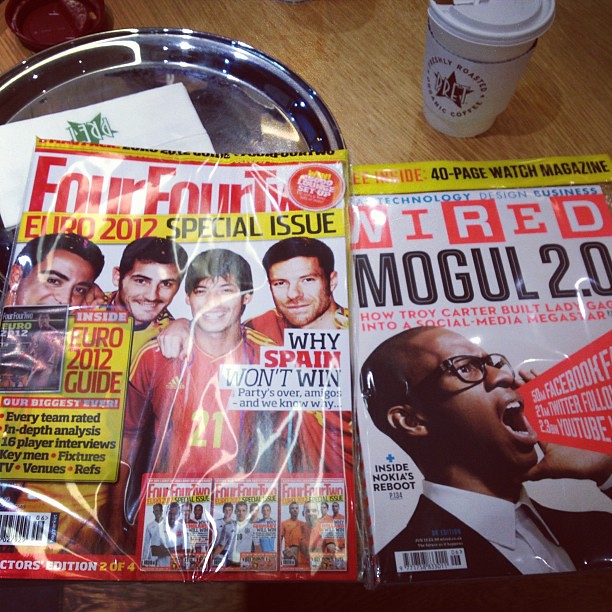This image, a square color snapshot taken from above with a flash, captures a tabletop scene with two prominently displayed magazines still in their original plastic packaging. The wooden table, a light brown color, is set diagonally across the frame. Both magazines occupy most of the image, with the left magazine showing the title "4-4-2" in red text, promoting a Euro 2012 special issue with a yellow square highlighting key features like team analyses and fixtures. The magazine cover features a group of smiling individuals in jerseys with the headline "Why Spain Won't Win." The right magazine, titled "Wired," features a cover story on Mogul 2.0, detailing how Troy Carter built Lady Gaga into a social media megastar, with images emphasizing her massive following across various platforms.

Behind the left magazine, a silver, round, and highly reflective platter is partially visible, with a white napkin adorned with green text and a logo that says PRET peeking out from under the magazine's corner. Above the right magazine sits a to-go coffee cup, white with a white lid, bearing a logo of the brand PRET: a red star with the words "freshly roasted, organic coffee." Glare from the flash or overhead lighting highlights the plastic-wrapped surfaces of both magazines, adding a sheen that reflects the light.